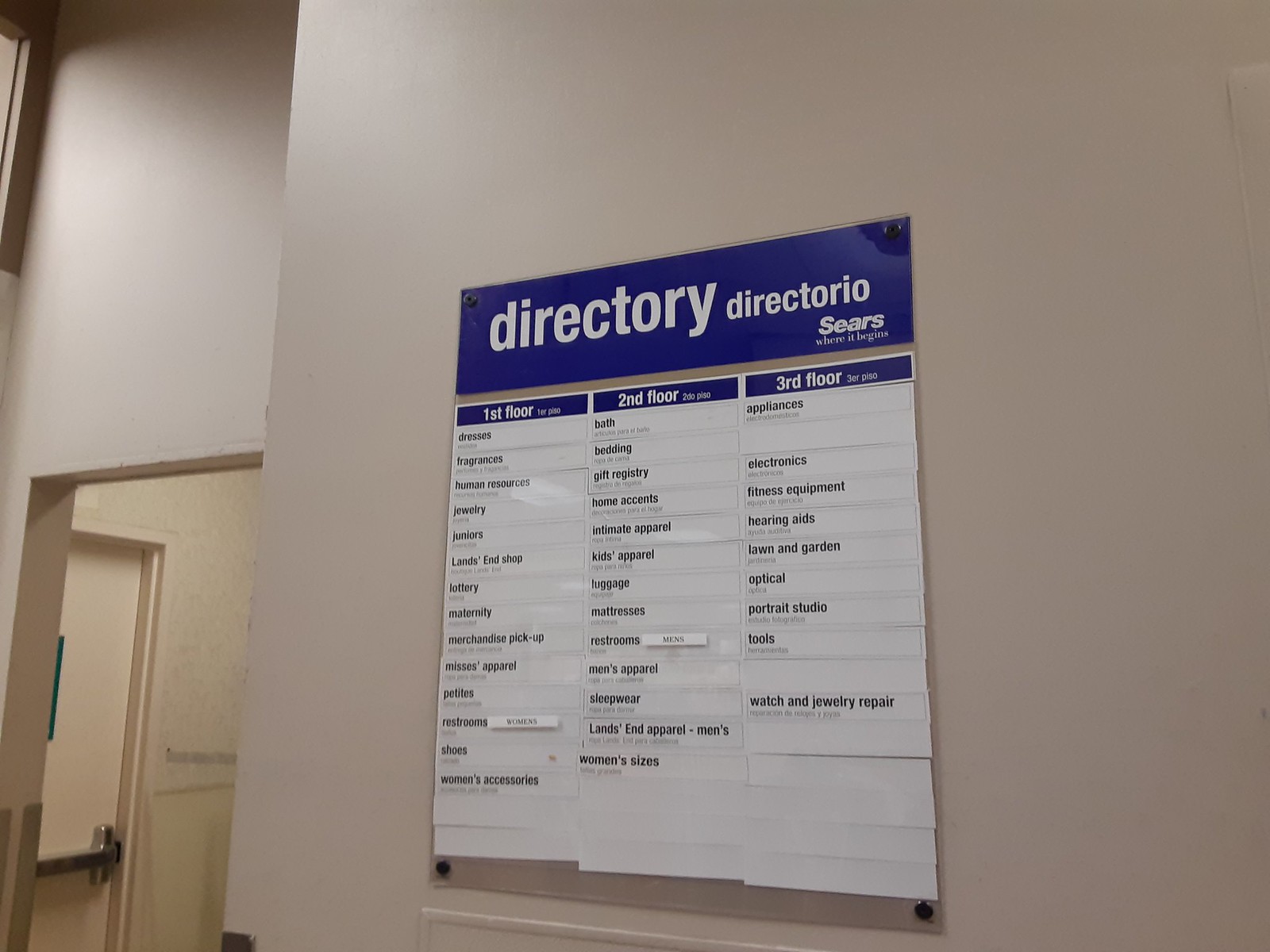The photograph features a directory prominently displayed against a tan-colored wall inside a department store. Adjacent to this wall is a doorway leading to another area with a similar tan door and light brown wall. This adjoining door appears to be a fire exit equipped with a silver metal push bar.

At the top of the wall-mounted directory is a blue rectangular sign labeled "Directory," introducing the information below. The directory itself is organized into three columns, each designated for a specific floor, and the text is presented in white color with black print.

The first column, labeled "First Floor," lists:
- Dresses
- Fragrances
- Human Resources
- Jewelry
- Juniors
- Land's End Shop
- Lottery
- Maternity
- Merchandise Pickup
- Mrs. Apparel
- Petite's
- Restrooms
- Shoes
- Women's Accessories

The second column, labeled "Second Floor," includes:
- Bath
- Bedding
- Gift Registry
- Home Accents
- Intimate Apparel
- Kids Apparel
- Luggage
- Mattresses
- Restrooms
- Men’s Apparel
- Sleepwear
- Land's End Apparel
- Women’s Sizes

The third column, designated "Third Floor," provides:
- Appliances
- Electronics
- Fitness Equipment
- Hearing Aids
- Lawn and Garden
- Optical
- Portrait Studio
- Tools
- Watch and Jewelry Repair

This detailed directory serves as a comprehensive guide for shoppers navigating the department store.